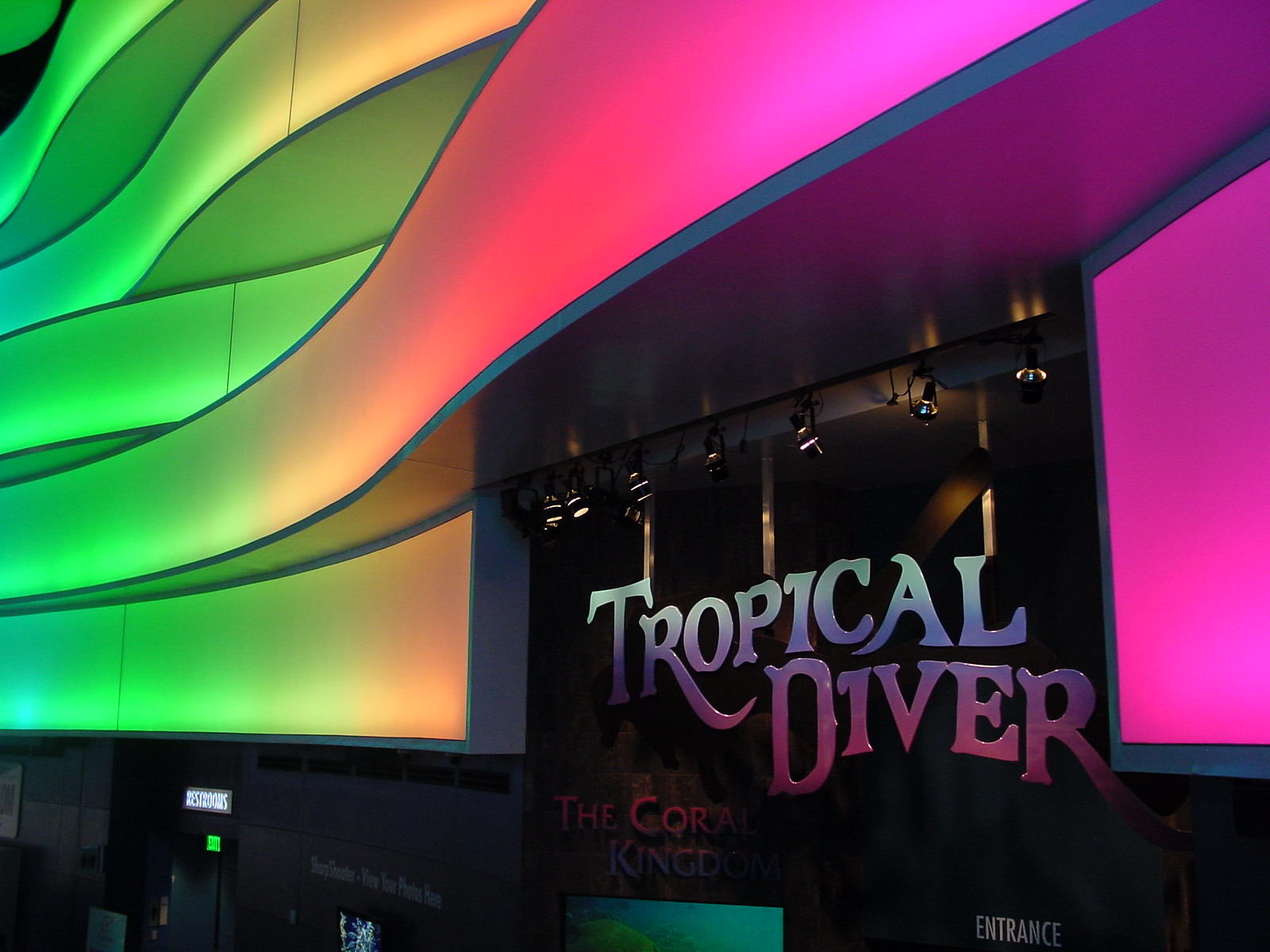The image depicts the entrance to an aquarium attraction called "Tropical Diver: The Coral Kingdom." The vibrant exterior features iridescent colors with the text "Tropical Diver" transitioning from light blue to pink, set against a backdrop of tiered wave-like designs in green, pink, and blue. Beneath the "Tropical Diver" text, "The Coral Kingdom" is prominently displayed. On the right side, there's a stage-like setup with curtains and floodlights, giving the appearance of an underwater world. The building facade has bright pink and yellow tones, creating a colorful and inviting atmosphere. To the left, a "Restrooms" sign in bright white letters is visible, indicating the facilities available to visitors. Confusingly, it appears both the interior and exterior elements of the entrance are captured, with doors marked "Entrance" located in the bottom right corner. Overall, the image conveys a lively, marine-themed setting, with underwater motifs and colorful decorations.